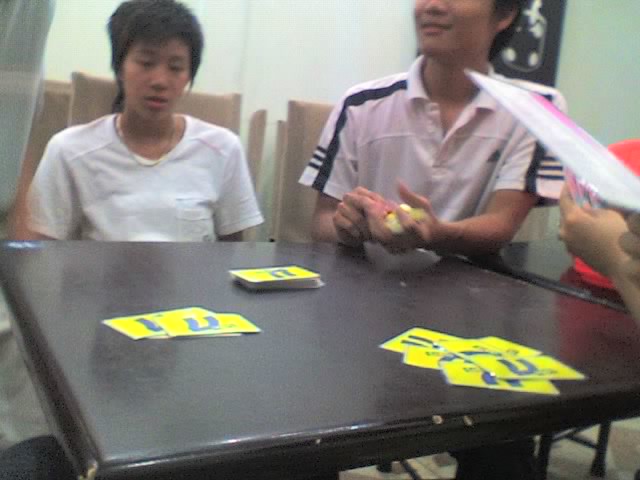Three friends gather around a square black table to enjoy a game of cards. The seating suggests the presence of a possible fourth person, as the individual on the middle-right is smiling and looking beyond the frame. The person on the left, dressed in a white short-sleeved shirt, gazes intently at the table. Meanwhile, the person on the right, also in a white short-sleeved shirt but with distinctive black piping, is skillfully shuffling a deck of cards. The cards are predominantly yellow with a blue design in the center, though the exact details of the design remain unclear. To the lower left and right of the table lie separate piles of cards, with the main deck neatly stacked in the center. The person at the far right, of whom only the hands are visible, holds what might be a scorecard or the game’s rules. The atmosphere is genial, accented with smiles, indicating a pleasant camaraderie among the group. The image captures a moment of friendship and casual leisure, underlined by their collective engagement in the card game.